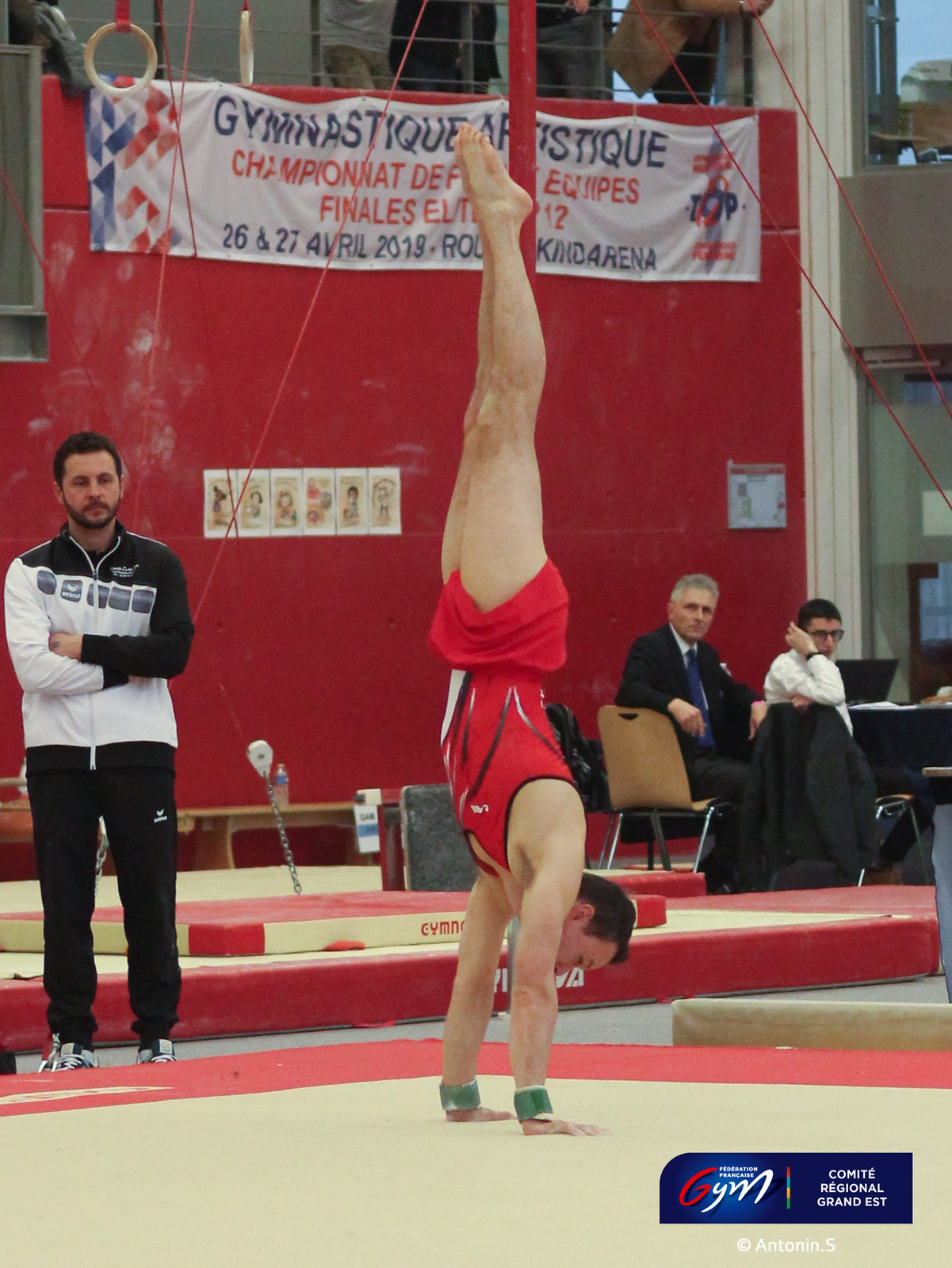In an indoor gymnastics arena, a gymnast is showcased performing an impressive handstand at the center of the image, perfectly straight with toes pointed upward. The athlete is attired in a vibrant red tank top and matching red shorts, with green wrist wraps visible. They are positioned on a tan mat surrounded by a red border, against a backdrop of a red wall adorned with a prominent white banner. The banner reads "Gymnastique Artistique" in blue text, and "Champion Finals Élite" in red text, with additional details partially obscured, indicating a championship event. To the left of the gymnast, a man dressed in a black and white tracksuit, likely the coach, stands observing the athlete. On the right side of the image, two men seated at a desk appear engaged, watching the performance closely.